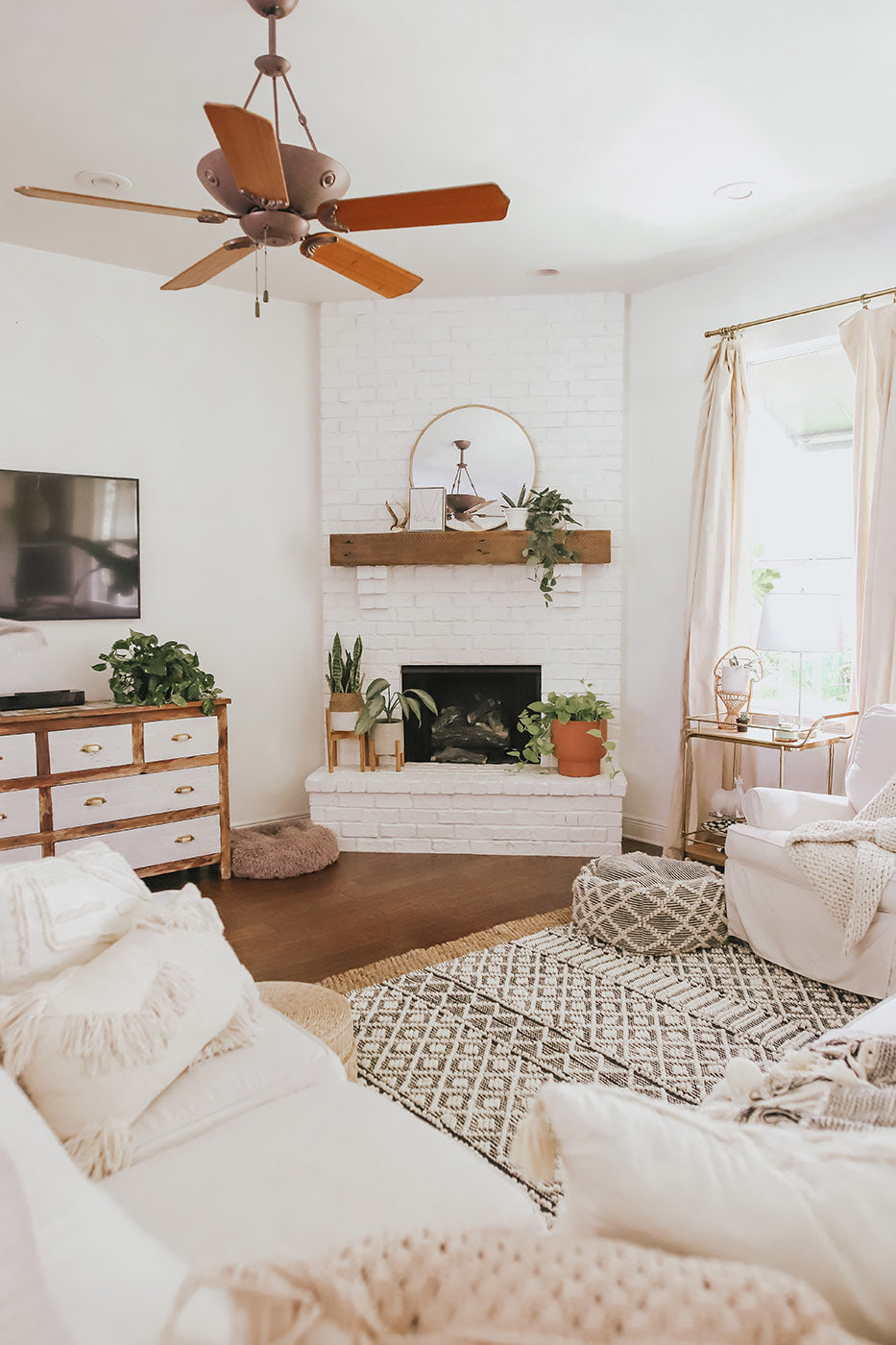This color photograph, taken in portrait orientation, captures the clean and bright interior of a Scandinavian-styled living room. The room is predominantly decorated in various shades of white, with minimal but striking wooden accents that enhance its modern and airy aesthetic. The walls and ceilings are completely painted white, providing a crisp and serene backdrop.

In the center of the image, a corner fireplace, adorned with a mantle of dark wood, stands out against the white stone bricks. It is decorated with soft wood pieces and topped with a round mirror. Below the fireplace are some plants, adding a touch of greenery to the minimalist decor.

On the left side, a white chest with dark wood trim and white door fronts sits under a panel TV mounted on the wall. A terracotta planter adds a splash of color next to it. Above everything hangs a pendant-style ceiling fan with five dark wooden blades, serving as an elegant accent piece.

The room features a large beige rug with a brown checkerboard pattern in the middle, tying the space together. In the foreground, the soft arm of a white sectional sofa adorned with throw pillows and blankets is visible on the left. To the right, there's a white overstuffed chair with a slipcover beside a round ottoman. A tea cart stands near a window to the right, with long vertical drapes drawn open to let in natural light.

This well-maintained and thoughtfully designed room emphasizes comfort and simplicity, incorporating woven, linen, and fringe items that give it a slightly bohemian touch, while still maintaining the clean lines and muted palette characteristic of Scandinavian design.